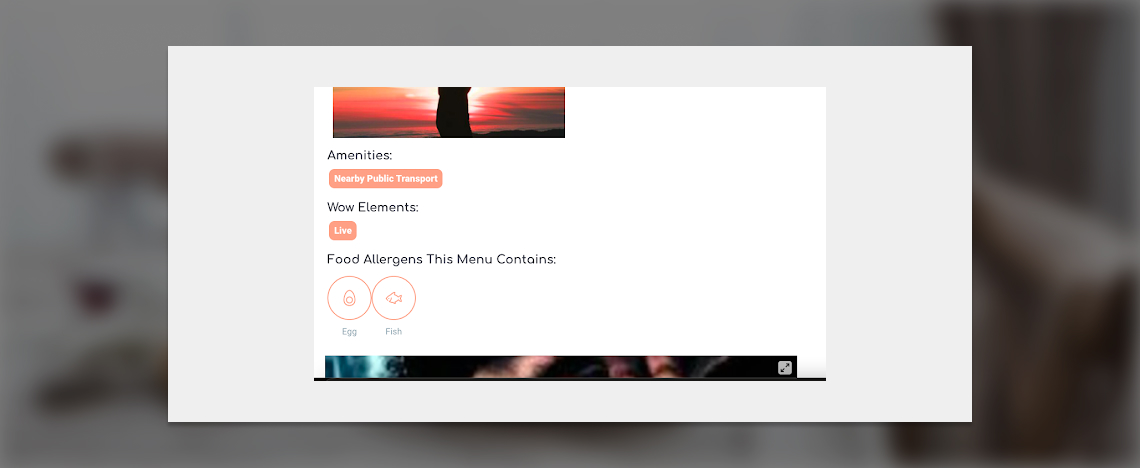The image presented is a screenshot likely taken from a restaurant's digital menu or information board, characterized by a densely packed array of details within a short, wide rectangular frame. The background is predominantly blurred to dark gray but features a discernible human elbow on the right-hand side, adding a touch of realism to the scene.

Central to this image is a tiered arrangement of boxes, each with specific contents. The main background houses a light gray box, which itself contains a smaller white box. Within this white box, the bottom half of a photograph is visible, depicting the hues of a sunset alongside the dark silhouette of a person, creating a striking visual contrast.

Below this image, black text reads "Amenities:" followed by a peach-colored rectangular box displaying "nearby public transport" in white letters. Continuing down, the term "Wow elements:" appears in black text, and beneath it lies another peach-colored rectangular box with the word "live" inscribed in white.

Further down, a heading in black text reads "Food allergens: This menu contains:" and is followed by two circular icons. The first circle, bordered by a thin peach outline, features the image of a halved boiled egg, with the word "egg" printed below it in medium gray letters. Adjacent to this, the second circle framed by a small peach-colored outline exhibits the outline of a fish, accompanied by the term "fish" in light gray lettering.

At the very bottom of the frame, there appears to be the beginning of another image. However, this additional picture is too blurred to discern any specific details, remaining an indistinct element within the overall composition.